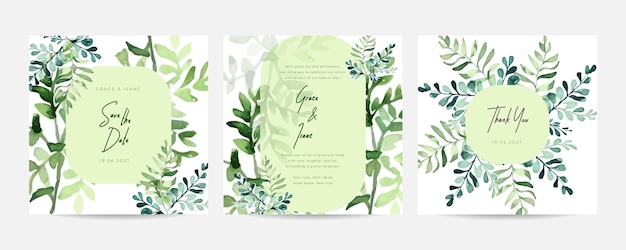This image is a narrow horizontal rectangular photograph displaying three equally sized note cards featuring botanical designs, each arranged side-by-side on a light gray background. The leftmost card showcases a light green rectangular panel in the center with unreadable dark green cursive text and a border accented with painted green leaves against a white background. The middle card features a similar design with an irregular oval-shaped light green panel bordered by green leaves; the panel includes the names "Grace and Isaac" in cursive text, although the date appears somewhat illegible. On the right, the card displays a circular light green panel enclosed by radiating green fronds, with the cursive text "Thank You" within the circle. Each card emphasizes a theme of white and green using watercolor-style leaf illustrations, contributing to an elegant, cohesive wedding stationery collection in a color illustration product photography style.